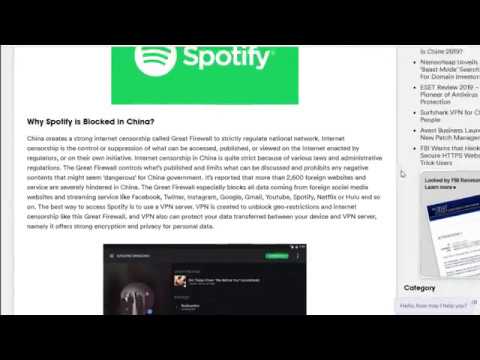The image is a screenshot featuring a series of distinct elements. At the top of the rectangular frame is a solid black banner. Directly below it, there is a green box with crisp white text displaying the word "Spotify." Beneath this box, the prominent black text on a clean white background poses the question: "Why is Spotify blocked in China?" 

Below this question, the image is filled with a substantial amount of blurry text where only a few keywords are legible, including "China," "Administration," "Foreign websites," "Best," "VPN," "Your device," and "Personal data." These words hint at the content that discusses the restrictions and possible workarounds regarding Spotify's availability in China.

At the bottom of the image, another black banner runs horizontally across the width of the frame. Positioned on the right side of the image is a gray box containing bold text that reads "Category." This layout suggests that the screenshot is part of an informational web page or article exploring the topic of internet censorship and the technicalities of accessing restricted content.